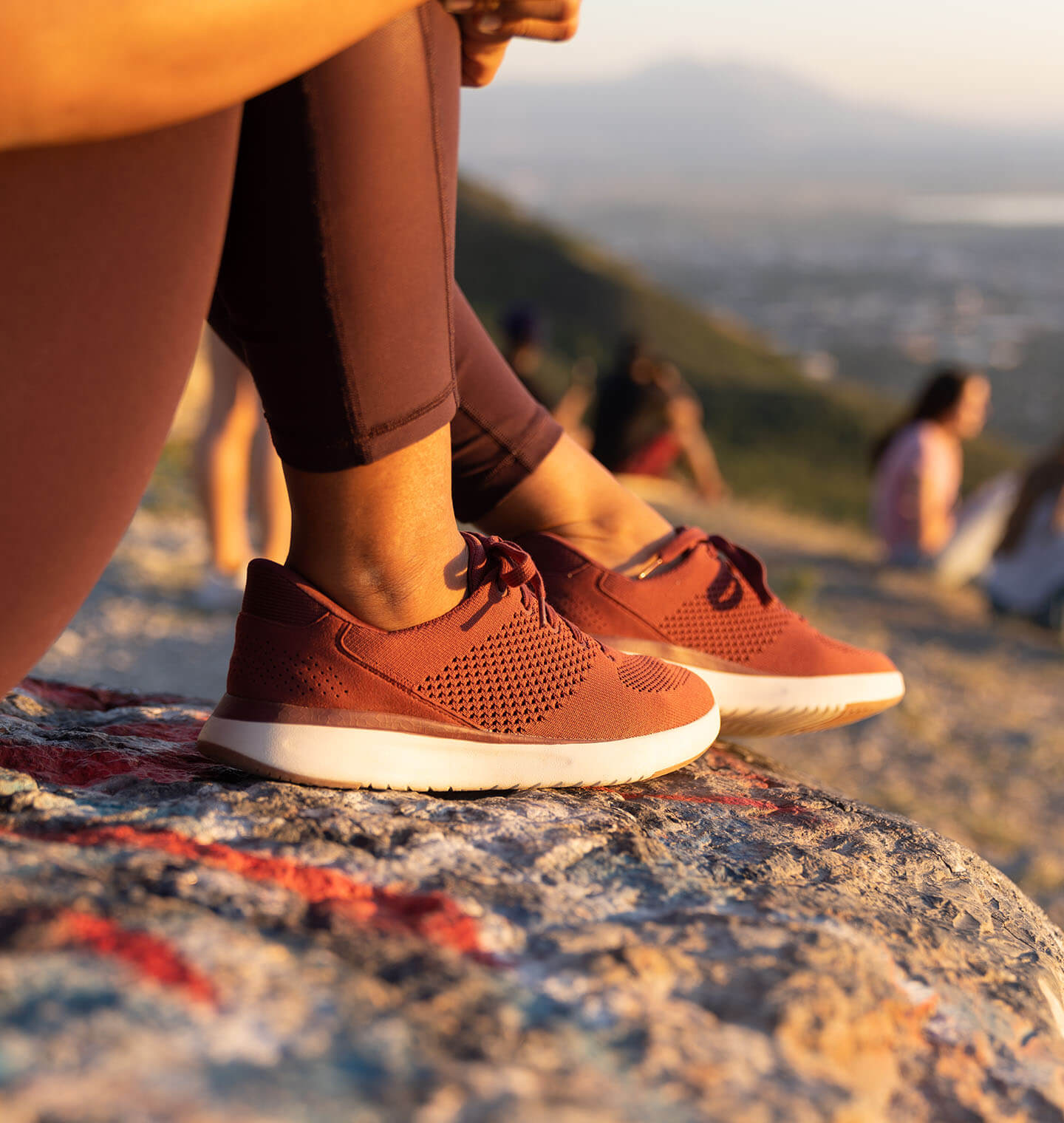The image depicts a close-up view of a woman sitting on the edge of a large gray rock with red markings, resembling graffiti or paint. Her legs are bent at the knees, and she is dressed in brown or black yoga pants and red or brown athletic sneakers with white soles. The photo primarily focuses on her lower legs, feet, and the backside of her thigh. There are several other people present in the scene, all sitting and somewhat out of focus in the background, contributing to a sense of depth. The surrounding area appears to be elevated, resembling a mountaintop or hillside, with a panoramic, foggy view of descending mountains and a blurry city or town in the distance. The coloration and lighting suggest it might be taken during daylight, possibly at sunset or golden hour. The overall setting evokes a peaceful, contemplative atmosphere with the woman and others seemingly engaged in relaxation or conversation while enjoying the scenic overlook.